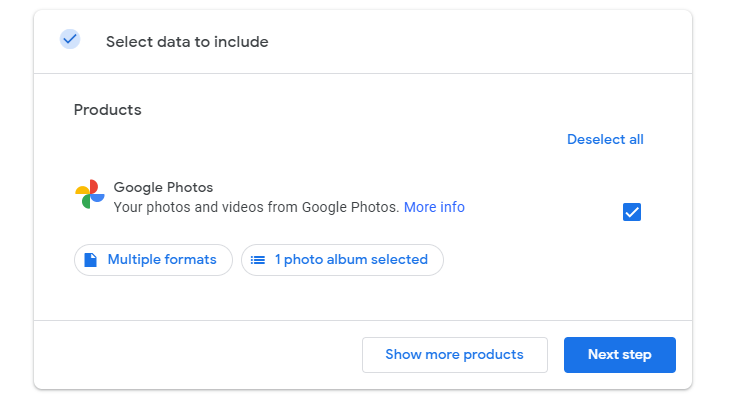This is a horizontally-oriented screenshot commonly seen on computer or smart device interfaces, providing details on customizable settings for data selection. The background is plain white, which highlights the interface elements. The image shows a gray-bordered window with rounded corners.

In the upper left corner, there is a light blue circle containing a dark blue question mark icon. Next to it, a bold black text reads "Select data to include." Below this header, a horizontal divider line separates the sections. Under "Products," to the right, a blue "Deselect all" option is available.

Further down, an icon representing Google Photos is visible, followed by the text "Google Photos." This section details that it includes "Your photos and videos from Google Photos," accompanied by a clickable "More info" link in blue. There is a blue-filled square with a white checkmark indicating selection.

The interface also displays multiple format options and notes that one photo album is selected. Another horizontal gray separator line is visible, and at the bottom, options for "Show more products" or "Next step" appear in blue, indicating further navigation possibilities.